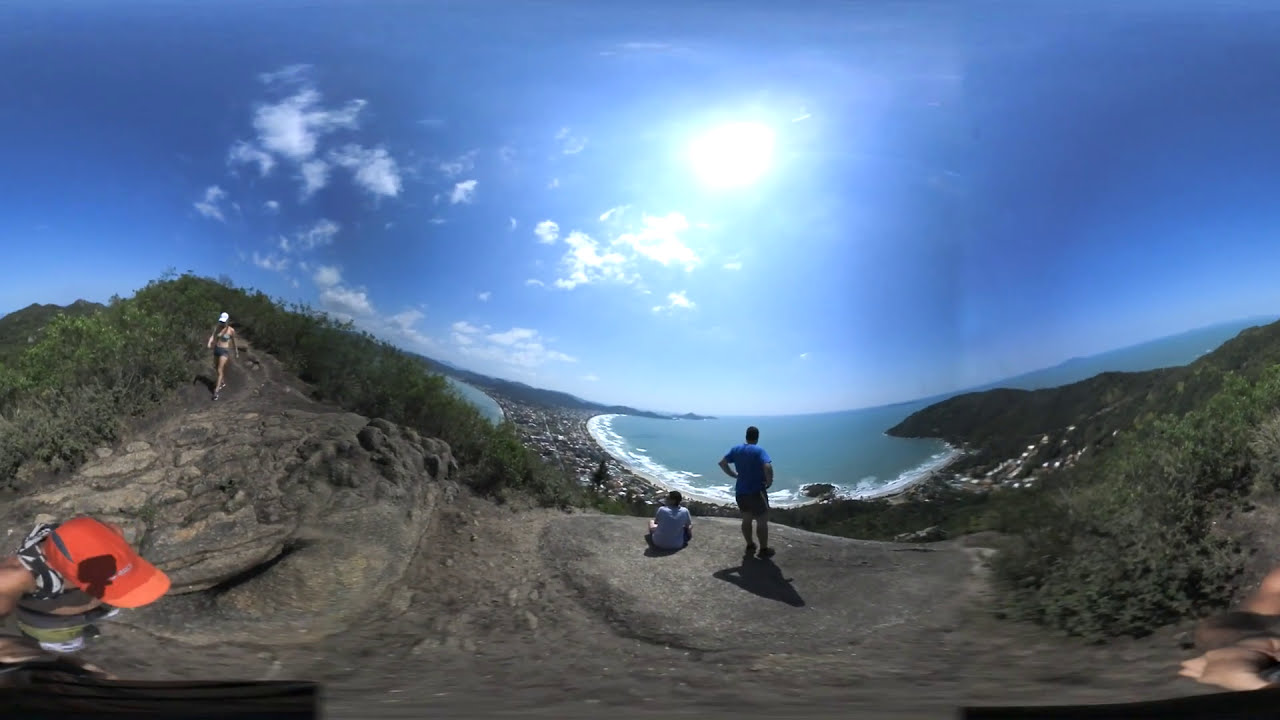This expansive panoramic photograph captures a scenic outdoor setting with four people positioned on a rocky, dirt-covered hillside that overlooks an ocean. Central to the image are two men: one standing and the other seated. The standing man, positioned to the right, is dressed in a blue t-shirt and dark shorts, gazing out at the teal-blue waters, where waves crash white against the distant shore. The seated man to his left wears a white t-shirt and grey shorts, blending into the stone outcropping they occupy.

To their left, or possibly behind them due to the panoramic distortion, a woman clad in a bikini top, shorts, and a white cap is seen climbing down the hill. The blurry presence of another person is barely discernible in the upper left corner, featuring an orange hat and a green outfit with a black and white backpack, who might be the photographer.

The backdrop of this vivid landscape includes green trees and bushes set against a blue sky with white, wispy clouds. Below the rocky prominence, the coastline is adorned with hints of grass and sandy zones as the ocean meets the shore. The image, with its wide-angle lens effect, captures a serene moment of nature observed from a high vantage point.